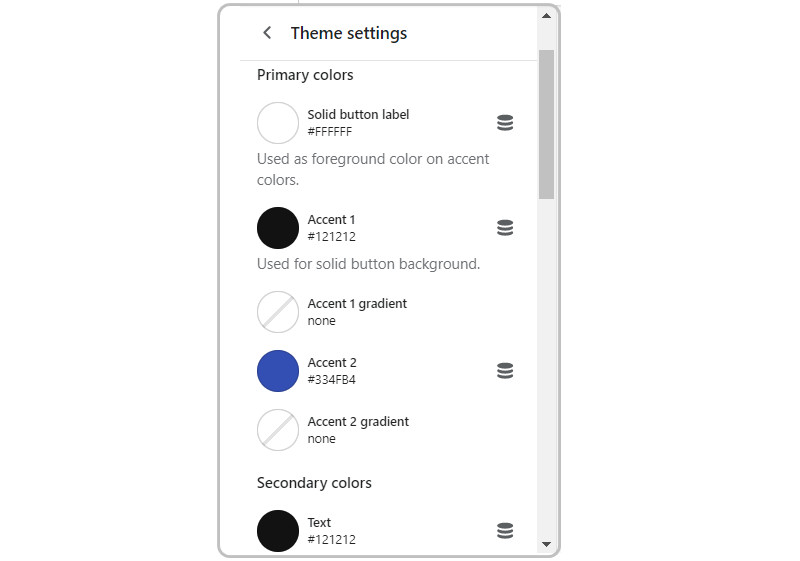The image depicts a white, rounded rectangle pop-up box with a 2-3 pixel border. The header of the box reads "Theme Settings" in black text, set against a white background with gray accents. The primary color is set to hex code #FFFFFF, representing a solid white used as the foreground color for accent buttons. To the right of each color setting is a small button, presumably allowing the user to modify the color. 

Additional settings include:
- Accent 1: Hex code #121212, a dark gray almost black, used for solid button backgrounds. The gradient for Accent 1 is set to 0.
- Accent 2: Hex code #334FB4, a dark blue. The gradient for Accent 2 is set to none.

The secondary color and text setting are both set to hex code #121212, matching the dark gray of Accent 1, almost the darkest shade without being black.